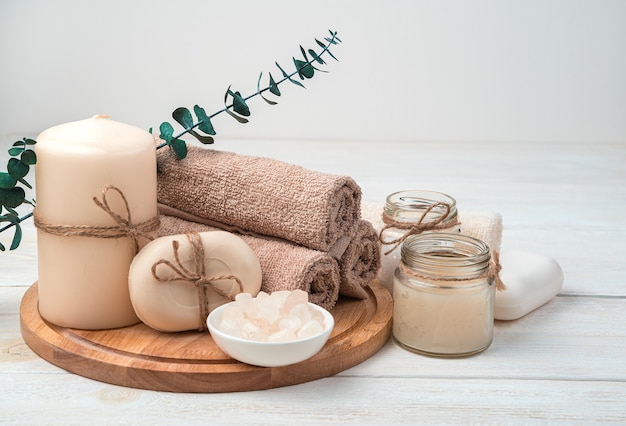This tranquil image showcases a beautifully arranged display of spa products set against a white wooden table background. Central to the composition is a circular wooden board that holds a selection of self-care items. Resting on the board is a small white bowl containing light pink round objects, possibly bath salts or large dissolvable stones, accompanied by a neatly wrapped bar of peach-colored soap with a light brown twine. A matching peach candle, also adorned with the same light brown twine, stands behind the soap. Flanking them are three rolled-up towels, which vary in shades of tan, beige, and a darker peach color. Enhancing the serene ambiance further, other items include two smaller white candles in glass jars positioned off the wooden board. Completing the spa-themed scene, a sprig of greenery, possibly eucalyptus, extends into the background, adding a natural touch to the meticulously styled setup. The overall aesthetic exudes a sense of calm and relaxation.